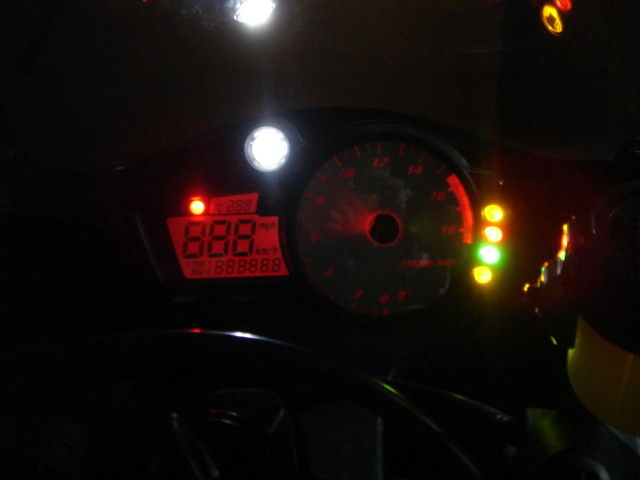The image is a landscape-oriented photograph dominated by a very dark black background. At the very top, a white light is positioned towards the center, accompanied by a reddish light on the right-third area. In the center of the image, a dimly lit tachometer stands out, featuring red numbers arranged in a circular fashion. On the far right of the tachometer, a solid red bar spans the final two numbers, indicating the tachometer's maximum range. The pivot point is marked by a central circular hub.

To the left of the tachometer, there is a digital display. This display prominently shows '888' in large black numbers on an orangish-red background. Above this main reading, there's another red light placed over the first digit '8'. There is also an adjacent white display. Below the '888', smaller digits likely indicate the mileage. On the right side of the tachometer, there are four vertically aligned indicator lights; the sequence from top to bottom includes two yellow lights, one green light, and another yellow light.